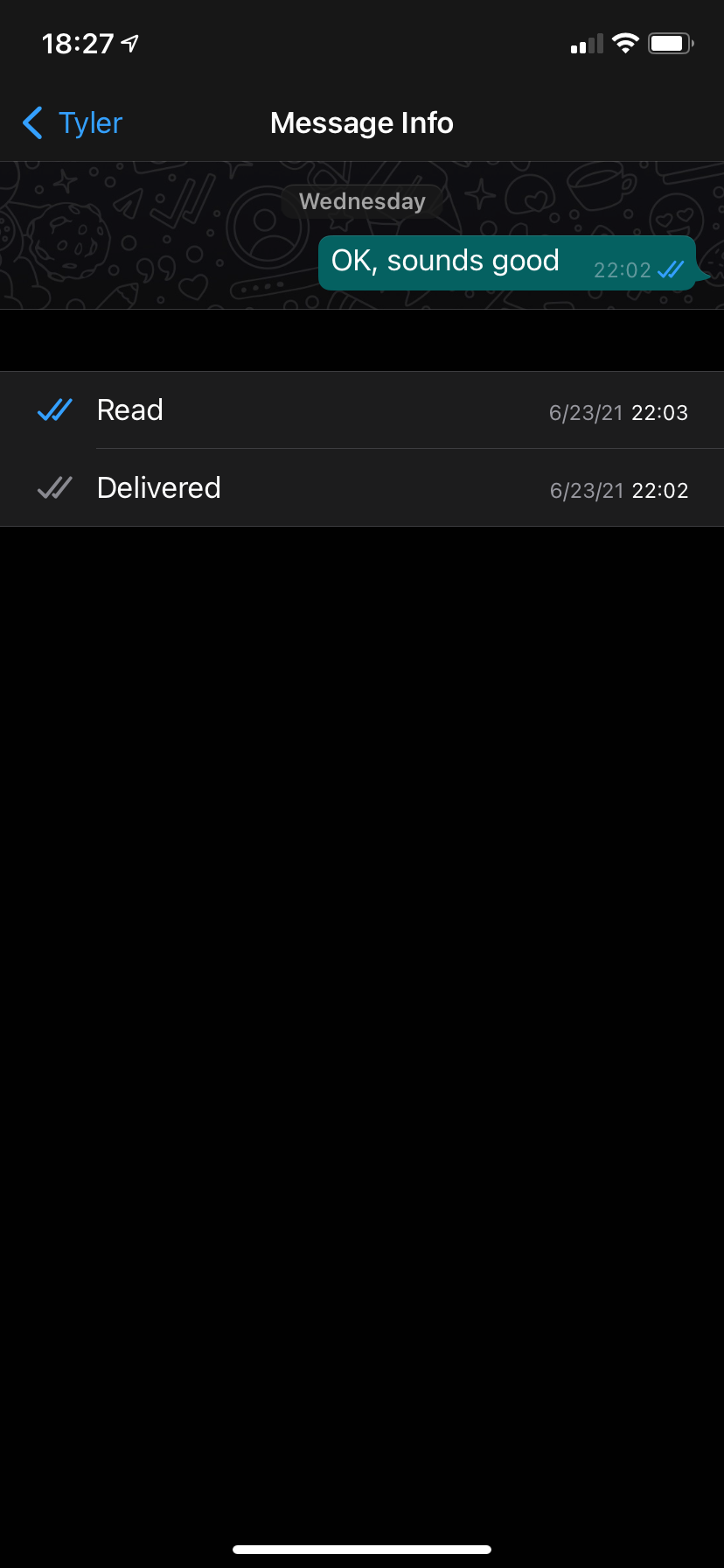This screenshot captures a smartphone screen displaying a messaging application interface. The background is predominantly black with minimal elements. The current time is shown as 18:27. A prominent blue arrow pointing to the left beside the name "Tyler" indicates that the message is from Tyler. The screen features a heading labeled "Message info," and directly below it, the day "Wednesday" is displayed.

The main content includes a message from Tyler that reads, "Okay, sounds good." This text appears on a turquoise banner, indicating that it was sent and subsequently read. According to the timestamps, the message was sent at 22:02 and marked "Read" at 22:03 on the 21st of June, 2023. The read receipt is confirmed by two small turquoise ticks adjacent to the "Read at 22:03" timestamp. Just above, a small grey banner indicates that the message was delivered at 22:02 on the same date.

With the exception of a narrow white bar at the bottom of the screen, likely for text input or navigation purposes, the remainder of the screen remains blank.